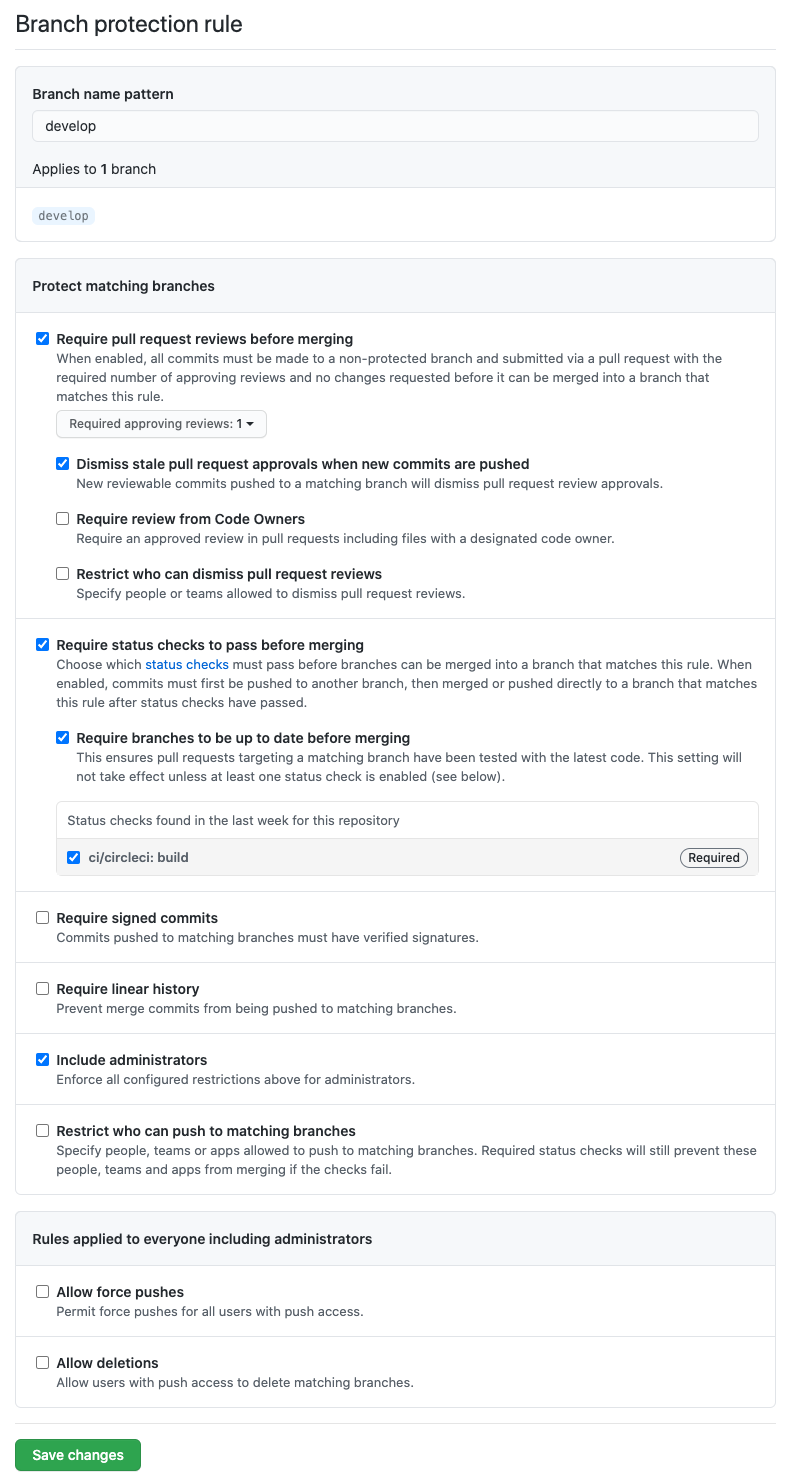This is an image of a branch protection rule settings screen on a cell phone. The screen primarily features black text on a white background, with some elements highlighted in faint gray to emphasize specific sections. At the top, the title "Branch Protection Rule" is displayed prominently. Below this, there's a gray rectangular box containing a white label with the word "develop," indicating the branch name pattern. 

This is followed by text stating "Applies to one branch" with the specific branch named "develop" clearly spelled out. Further down, the screen lists various protection options such as "Protect matching branches." 

Notably, there are several blue check marks indicating selected options. These include "Require pull request reviews before merging" and "Dismiss stale pull request approvals when new commits are pushed," among others. As you continue scrolling, some options are checked, while others remain unchecked.

At the very bottom, there is a green-gray rectangular button labeled "Save Changes," enabling the user to apply the configured settings.